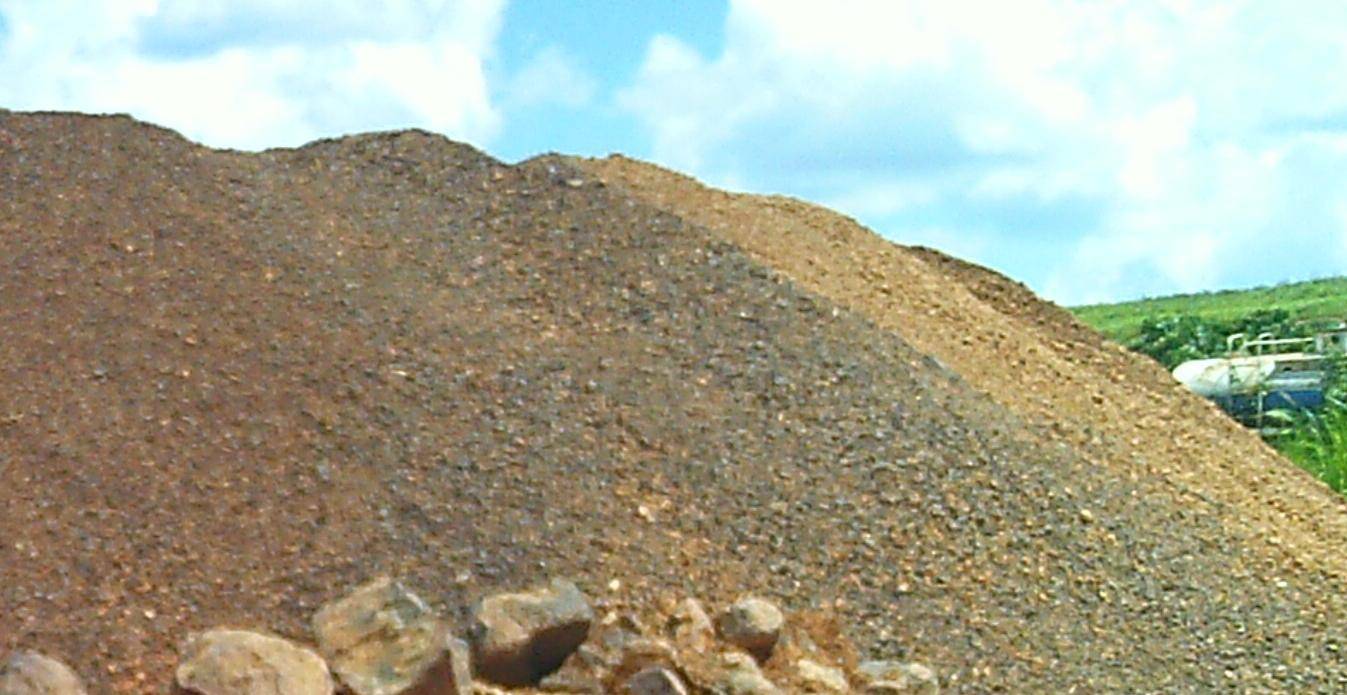This color photograph captures a scene dominated by an artificial mound of dirt, situated slightly to the left of the frame. The dirt, which exhibits hues of brown, orange, and black, appears to have been recently bulldozed into a substantial hill. In the foreground, a collection of sizable rocks is scattered from the left to the center bottom, primarily brown with some gray and black tones. To the right of the dirt mound, a green grassy area extends into the background. Visible behind the mound, there's a white tank equipped with metal railings and a stairway, suggesting an industrial setting, possibly a filtration system or treatment plant. Above, the sky is a vivid blue, adorned with white clouds that span across the upper quarter of the image.